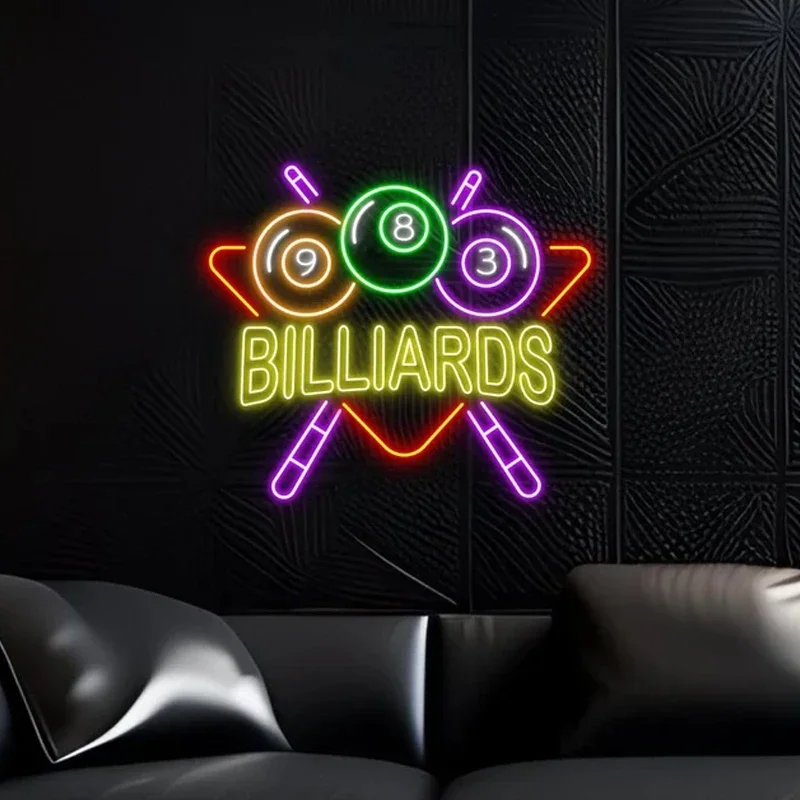The image captures a sleek, modern living space centered around a black leather couch, which features two leather pillows. Positioned against a textured black wall with a square tile pattern, directly above the couch, is an eye-catching neon sign dedicated to billiards. The neon sign prominently features the word "billiards" in yellow bubble letters, outlined in yellow, and is accentuated by an orange upside-down triangle, resembling a pool ball rack. Adding to the billiard theme, two purple pool cues cross behind the triangle. Topping off the design, three neon pool balls are displayed above the word "billiards": an orange 9-ball, a green 8-ball, and a purple 3-ball. The composition of the image draws focus to the vibrantly lit sign as the centerpiece of the setting.